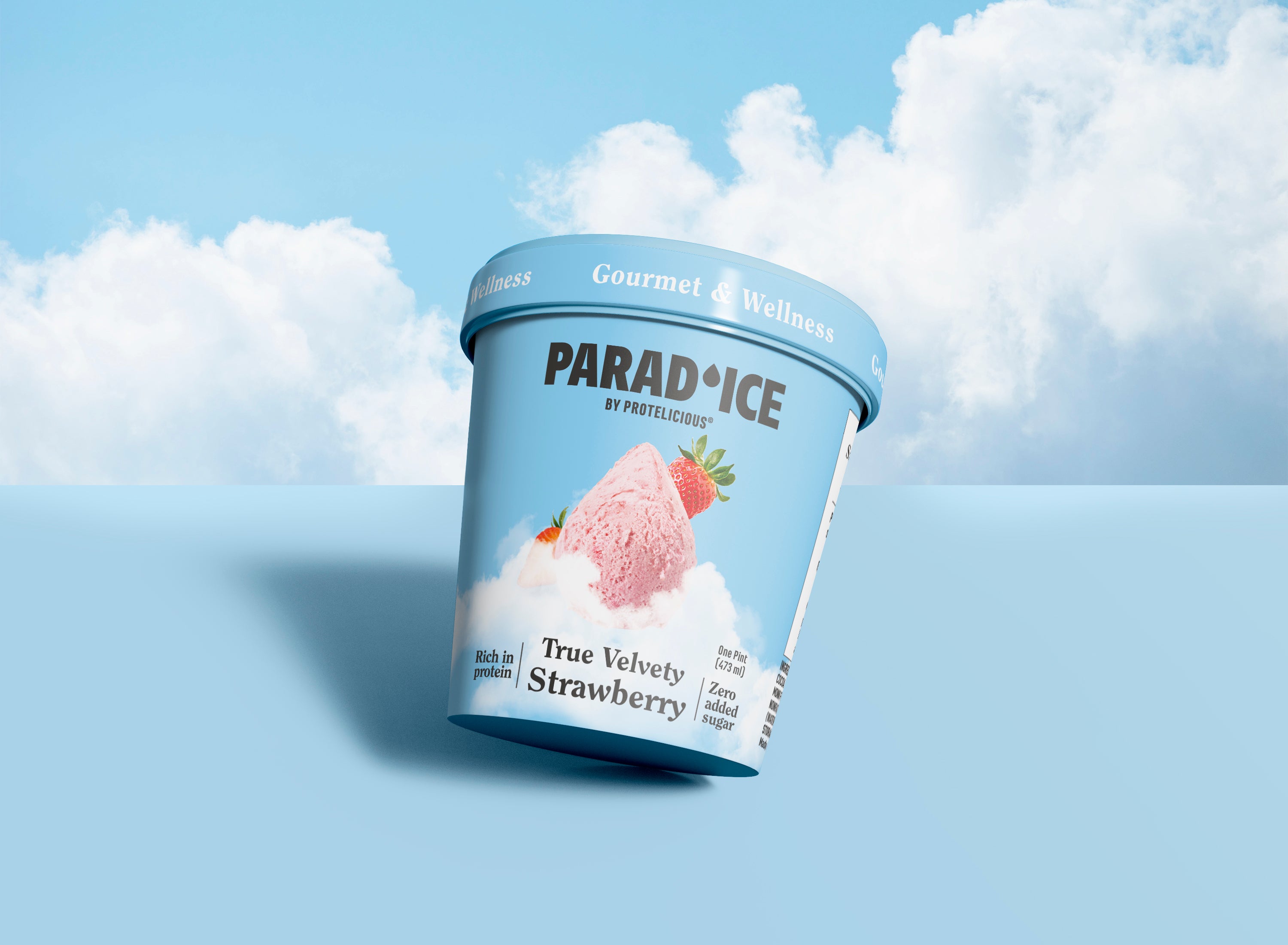This rectangular, horizontally aligned image showcases a visually appealing advertisement. The background is a vibrant sky with clear blue hues at the top and fluffy white clouds beneath, extending across the scene. In the foreground, a light blue table or counter surface mirrors the sky's color, creating a cohesive look. Centrally positioned on this surface, a pint of ice cream is tilted on its side, balancing delicately.

The ice cream container is predominantly blue and white. The rim of the lid is adorned with the words "Gourmet and Wellness" repeatedly printed in white. The brand name, "Paradise," is uniquely displayed with "P-A-R-A-D" in black and separated from "I-C-E" by a small water droplet, emphasizing the name creatively. Below this, the text "by Pro Delicious" or "by Pro-Talicious" (as variously mentioned) identifies the creator.

Central to the packaging design is a vivid image of a pink scoop of strawberry ice cream topped with a fresh strawberry, seemingly placed atop a gentle heap of clouds, enhancing the dreamy aesthetic of the product. Additional textual details on the container highlight the flavor, "True Velvety Strawberry," along with health-conscious notes such as "Rich in Protein" to the left and "Zero Added Sugar" to the right. The measurement "One Pint (473 milliliters)" is also featured, providing complete label information.